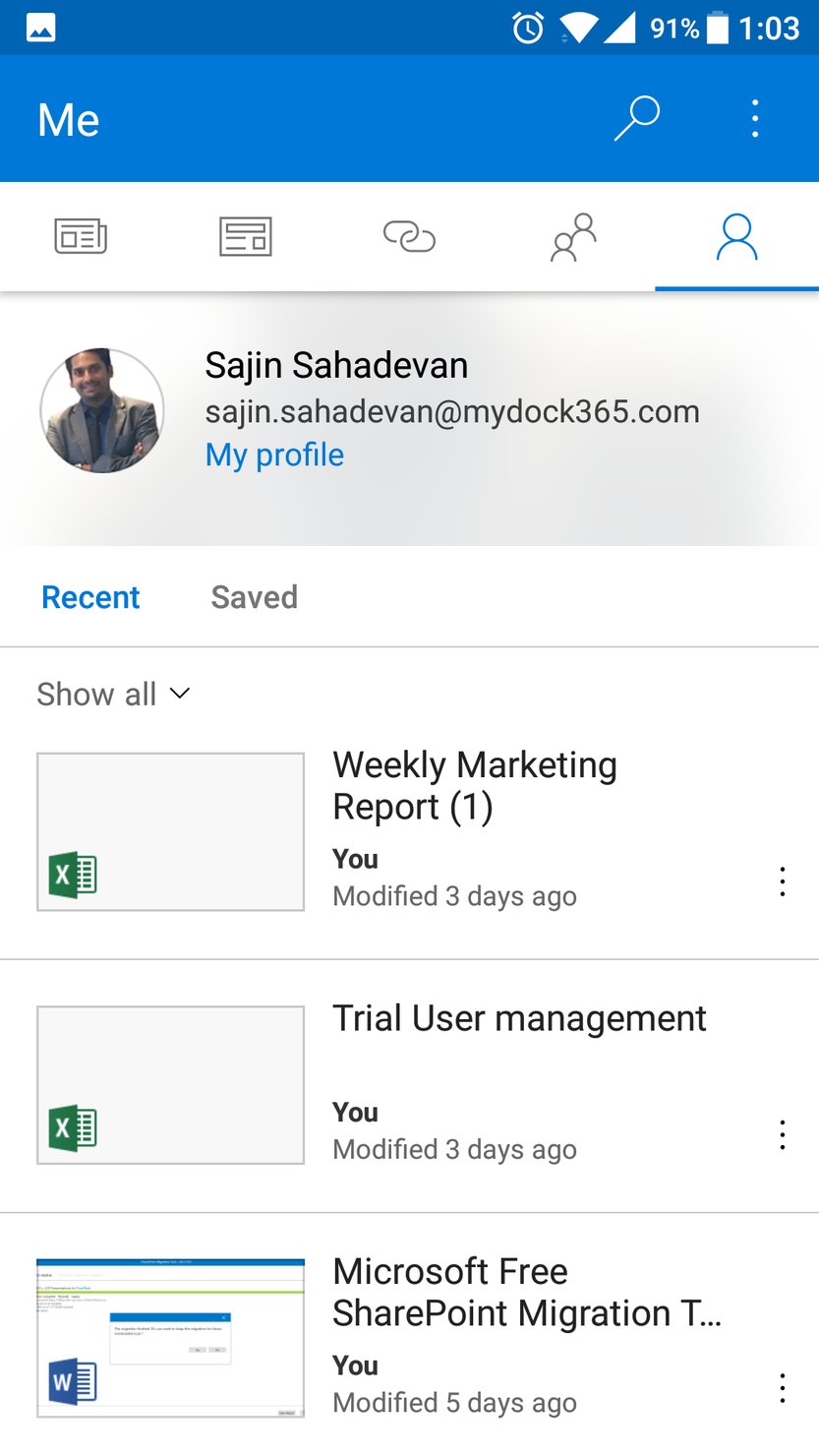The image showcases a detailed screenshot of a digital interface, likely from a communication or productivity app. At the very top, a blue header spans across the screen featuring a white square on the upper left side with what appears to be blue mounds inside it. On the right side of the header, a series of white icons are present: an alarm clock, Wi-Fi signal, reception phone service signal, and a battery icon displaying "91%." Additionally, the time "1:03" is visible in white.

Below the header, the interface transitions into a new level with the text "ME" in capital letters. Accompanying this text is a white magnifying glass icon and an arrangement of three white circles, aligned vertically. The background then changes to white where various symbols appear, including two newspaper icons on the left, two interconnected ovals, and a depiction of two black figures and another separate blue figure which is underlined in blue.

Further down, a gray background appears featuring a circular profile image of a man with brown skin wearing a gray suit. He is smiling with his arms folded. Next to the image, the name "Sanjan Sahadevin" is displayed, along with the email "Sanjan.Sahadevin@mydoc365.com." Below this, in blue text, "my profile" is indicated. The background reverts to white, highlighting the text "recent" in blue, signifying a clicked section, followed by "saved" in gray.

A thin gray line separates these sections, leading to a dropdown indicator labeled "show ordinance," represented with a black arrow pointing downward. The list beneath includes:
- "Weekly marketing report (1)" with the note "you modified three days ago."
- "Trial user management," also modified three days prior.
- "Microsoft free, SharePoint migration T..." which indicates it was modified five days ago.